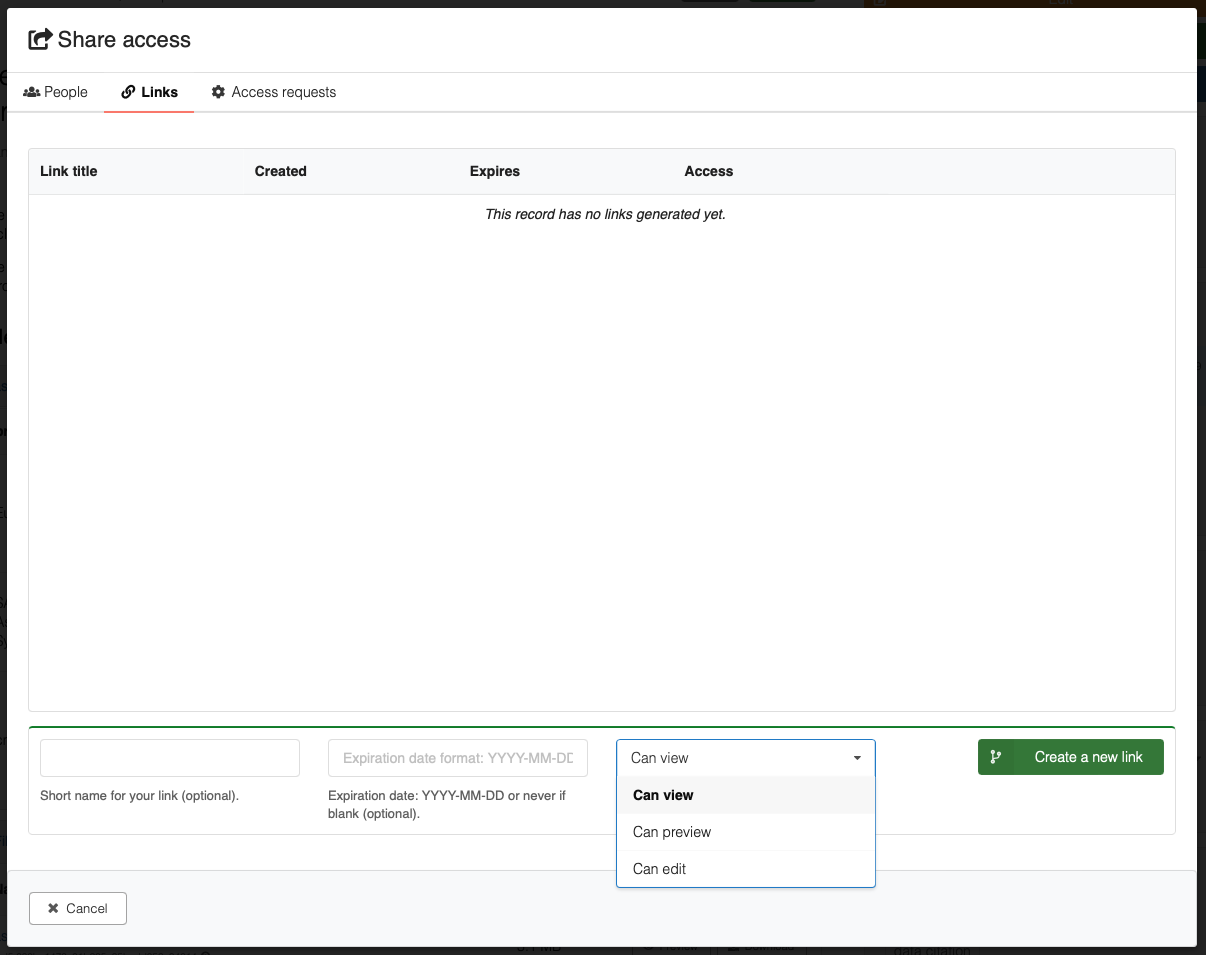The image displays a share access page with a slightly horizontal rectangular frame, bordered by a thin black line. The background of the page is predominantly white. In the top-left corner, there is a black share icon followed by the words "Share Access." Below this, three option icons are visible, representing "People," "Links," and "Access Requests." The "Links" option is highlighted, indicated by bold text and a red underline. 

Directly beneath, a chart format is presented with columns labeled "Link Title," "Created," "Expires," and "Access," but it currently shows no entries, with a message stating "This record has no links generated yet." 

At the bottom of the page, there is a dropdown menu with options "Can View," "Can Preview," and "Can Edit," followed by a prominent green button on the right labeled "Create a New Link."